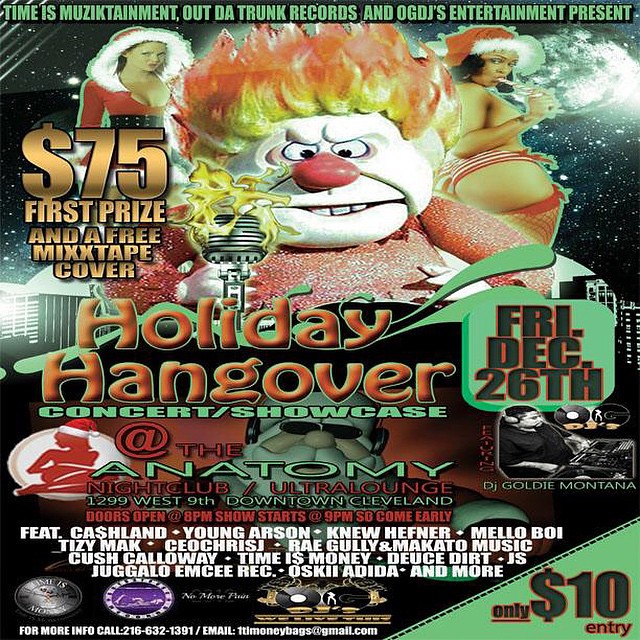This image is a large square advertisement poster for an event called "Holiday Hangover." At the very top, written in green all-caps text, it says, "Time Is Musictainment, Out Da Trunk Records, and OGDJ's Entertainment Present." Dominating the center of the poster is the title "Holiday Hangover," written in large orange letters.

The left side of the poster features a large gold dollar sign and the number "$75" indicating the first prize. Below it, also in gold text, it says, "First Prize and a Free Mixtape Cover." The event details below include "Concert/Showcase" in green text, and it specifies the location as "At the Anatomy Nightclub/Ultra Lounge, 1299 West 9th Street, Downtown Cleveland." In red text, the poster announces, "Doors Open at 8 p.m., Show Starts 9 p.m., So Come Early."

Towards the bottom, the featured artists listed in white text are Cash Land, Young Arson, New Hefner, and Mellow Boy. Additionally, in the lower right corner in a green triangular section, it states, "Only $10 Entry" in large black font.

Visually, the poster is striking with a black sky background filled with white dots representing stars. It depicts a woman on the left wearing a Santa outfit with a white fur hood, and near the center, a creepy clown figure with a big red nose, fiery hair, and an evil expression. To the right, another woman in a Santa hat and netted stockings is provocatively sucking on a candy cane, with part of her right butt cheek visible. This eclectic and detailed imagery creates a festive yet edgy atmosphere, emphasizing the unique vibe of the upcoming event taking place on Friday, December 26th.